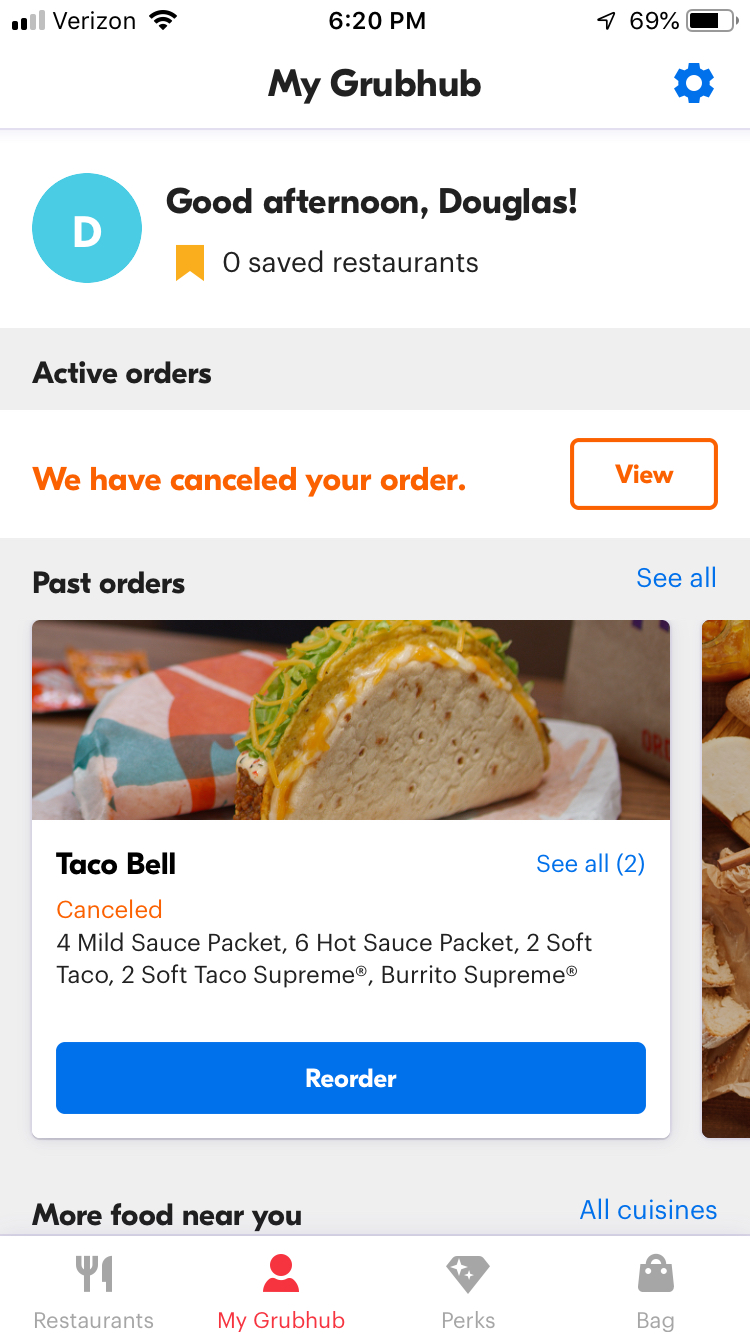The image is a vertical screenshot from a smartphone, capturing a moment within the Grubhub app. The background is primarily white, which is typical for many app interfaces. 

In the upper left corner, various status icons are visible, including:
- The signal strength indicator.
- The carrier information labeled "Verizon."
- The Wi-Fi signal icon.
- The current time, "6:20 p.m."
- The battery life icon displaying 69%.

Directly below these status icons, there is a blue settings icon. Centered on the screen in bold black text, it reads "My Grubhub." A thin line beneath this section serves as a separator.

Below the line, a blue circle with a white "D" inside it indicates the user's profile icon. The text "Good afternoon, Douglas" appears in bold black font. The interface indicates that there are "Zero saved restaurants" under this account. 

The "Active Orders" section shows a notification stating, "We have canceled your order," with options to "View" or select from "Past Orders." Specifically, a Taco Bell order was canceled, with an option to "Reorder."

At the lower part of the image, there are several navigational tabs labeled "More Food Near You," "Restaurants," "My Grubhub," "Perks," and "Bags." The "My Grubhub" tab is highlighted, indicating the current section displayed in the app.